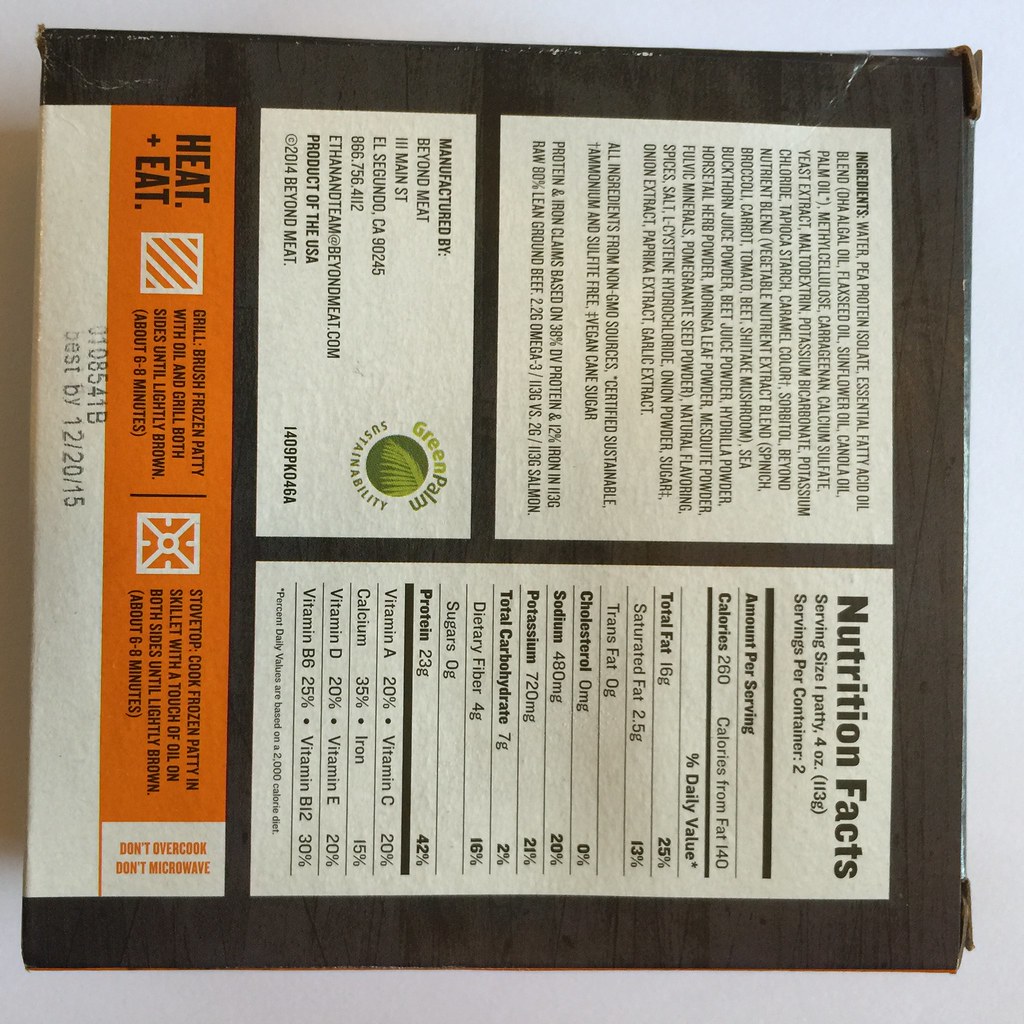The image depicts a nutritional label positioned sideways. At the very bottom, a red stripe contains the phrase "Heat + Eat," accompanied by additional, difficult-to-read text from this vantage point. Directly below this, warnings caution against overcooking and microwaving the product. At the very bottom, a number "0108541" and the letter "B" are displayed, along with an expiration date: "Best by December 20th, 2015."

At the top left corner of the label, there is a lengthy list of ingredients. Below the ingredients, it notes the manufacturer as Beyond Meat, located in El Segundo, California. To the right, the nutritional facts are provided, showing that the serving size is one patty (four ounces), with two servings per container.